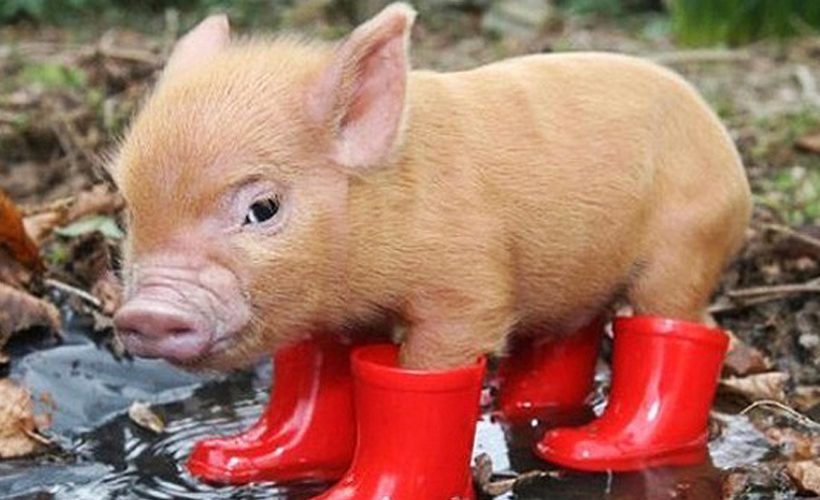In this delightful outdoor image, we see a close-up of an adorable little piglet standing in a shallow puddle surrounded by nature. The piglet, covered in light brown fur with pink ears and a pink snout, is donning four bright red rain boots on its feet, a thoughtful touch from its owner to keep its feet dry after a recent rainfall. The piglet’s single visible black eye peers curiously towards the camera, adding to its endearing expression, although it doesn't look too happy. The background features a mix of grass, leaves, twigs, and dirt, typical of a woodland setting, enhancing the natural atmosphere of the scene. This charming snapshot captures the piglet's innocent curiosity and the whimsical touch of its red boots against the earthy tones of its surroundings.